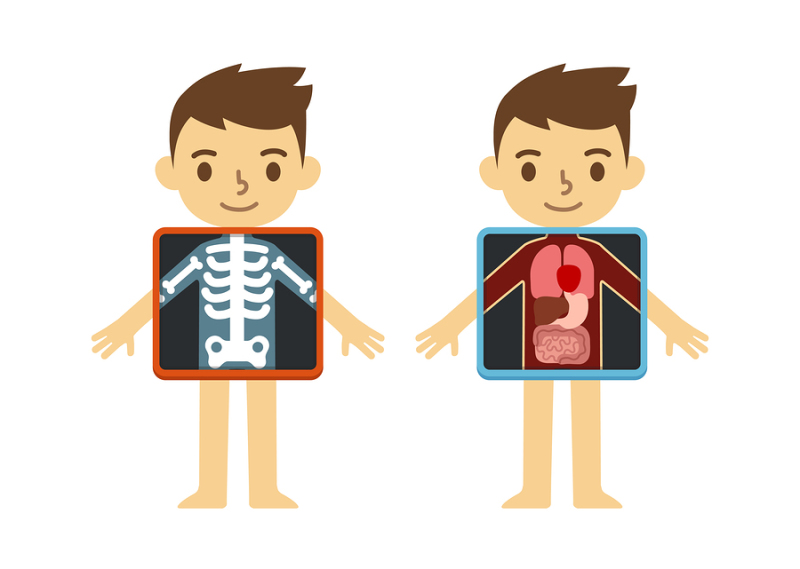This detailed cartoon-like vector drawing features two identical boys with wavy brown hair, both depicted without clothes and standing in front of x-ray machines. Each boy has their arms extended outward to the sides. The boy on the left is shown with his skeleton visible inside an x-ray monitor that has a red border and a black background. His skeleton includes the spine, ribs, humerus bones in the upper arms, and a simplified pelvis all interconnected. The boy on the right is displayed with a cutaway view revealing his internal organs inside an x-ray monitor framed in blue with a black background. Visible organs include his lungs, heart, liver, stomach, and both the small and large intestines. Both boys have light tan skin, gray-brown eyes, brown eyelashes, and light brown smiling mouths.